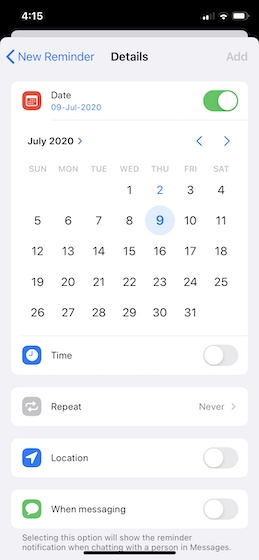Detailed Caption: 

The image is a screenshot captured on a mobile device, displaying a calendar app interface. At the very top of the screenshot is a black bar with white elements: the time reading 4:15 on the left, and the icons for battery power, Wi-Fi strength, and signal strength on the right. Just below this black bar, the app's interface begins with a simple pale grey background contrasted by white panels. 

In the top-left corner, a blue arrow pointing left is accompanied by the text "New Reminder" in blue. Centered at the top, in black text, the word "Details" is visible, while in the top-right corner, "Add" is written in very pale grey text.

Beneath this header section is a prominent white rectangle that comprises the main calendar view. This panel displays the month of July 2020, listing dates sequentially from Wednesday the 1st to Friday the 31st. Situated in the top-right corner of this calendar panel is a green oval slider with a white circle inside it, indicating an interactive element. Adjacent to this slider is a red square icon featuring a white calendar symbol.

At the bottom right of this calendar panel, a blue square icon with a white clock symbol is displayed, next to the black text reading "Time." 

Immediately below the calendar, another panel hosts a grey square icon presenting a circular repeating arrows symbol. To its far right, the text reads "Repeat" with "Never" in very pale grey text alongside a right-pointing arrow, denoting a default setting.

In the panel directly below, a blue icon featuring a compass arrow pointing towards the upper right corner is displayed, labeled with the text "Location." Beneath this is another section that contains a green icon with a speech bubble symbol, alongside the text "When Messaging."

At the very bottom of the image, pale grey text provides additional information: "Selecting this option will show the reminder notification when chatting with a person in Messages."